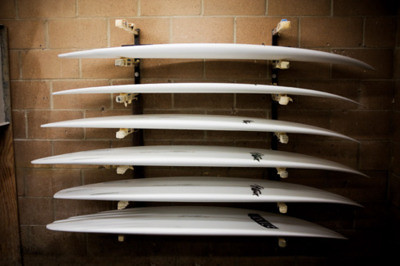This image features a vertically mounted rack on a large, reddish-brown brick wall with light gray grout. The rack, likely made of black iron, is bolted to the wall and consists of seven slots or shelves, though six are in use. Each shelf holds a white surfboard, which becomes progressively larger from top to bottom. The surfboards have a uniform design with black markings or logos, predominantly placed towards the middle or end of the boards. The surfboards, in pristine condition, suggest they may be in a repair shop or storage area. The right side of the image is darker, potentially indicating a shaded portion of the wall or a smaller, darker space within the shop. The left side faintly hints at additional shelving or storage, though it’s not clearly visible.